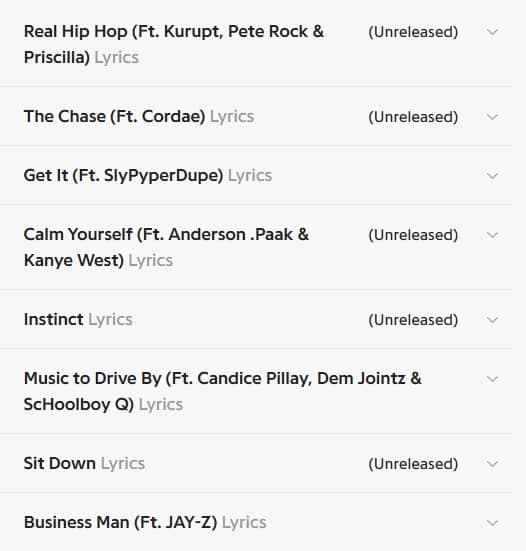This is a screenshot displaying rows of detailed information, seemingly cropped from a larger screen with a light gray background. Each row consists of bold text indicating song titles, followed by a lighter gray label that says 'lyrics.' On the right of each row, there is a medium gray arrow pointing downwards. To the left of these arrows, some rows include medium gray text in parentheses, indicating that the songs are 'unreleased.'

The entries are as follows:

- "Real Hip Hop (Ft. Kurupt, Pete Rock, and Priscilla)" indicated as unreleased.
- "The Chase (Ft. Cordae)" indicated as unreleased.
- "Get It (Ft. Sly Piper Dupe)"
- "Calm Yourself (Ft. Anderson .Paak and Kanye West)" indicated as unreleased.
- "Instinct," indicated as unreleased.
- "Music to Drive By (Ft. Candice Palet, Dem Joints, and Schoolboy Q)"
- "Sit Down," indicated as unreleased.
- "Businessman (Ft. Jay-Z)"

Each section is separated by a thin light gray horizontal line stretching across the width of the screen, though these lines fade out before reaching the right edge of the frame. The 'featuring' text is consistently written as 'Ft.' with a capital 'F' and a lowercase 't' followed by a period.